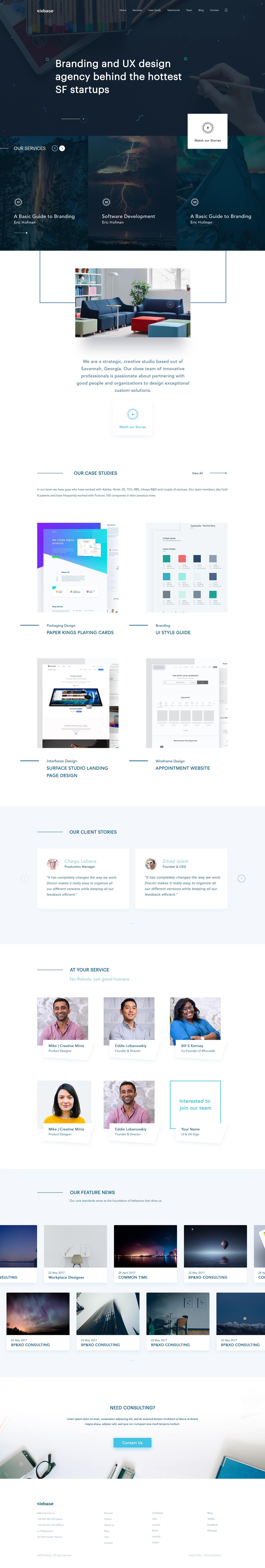The screenshot depicts a cell phone screen displaying an interface that appears to be from a website. At the top, there's a noticeable black bar which contains some images that are too dark to discern clearly. Below this bar, in the upper left corner, some white font is visible but not legible, while a larger white font in the middle reads: "Branding and UX design agency behind the hottest SF startups."

On the right-hand side, there's a white rectangle containing gray text, accompanied by a gray circle, though the specific text is unreadable. Directly beneath this, there is an image of a living room that features a blue couch and some windows to the right. Underneath the living room image, there is an extensive amount of gray text that is too small to be read clearly.

Furthermore, there are several sections of text and open windows suggesting design layout options or color selections for furniture. The background shifts to gray with two white text boxes that possibly contain customer testimonials. Beneath this is a 3x2 grid of pictures; the top row includes images of three people: an African American man, a Caucasian man, and an African American woman. The second row contains a Caucasian woman, a person of darker complexion, and a box of text that is unidentifiable. Following these images are various other pictures that are mostly illegible.

At the bottom of the screen, there is a blue button, presumably for navigation or a call-to-action, followed by a considerable amount of gray text that is so small it appears as indistinct squares.